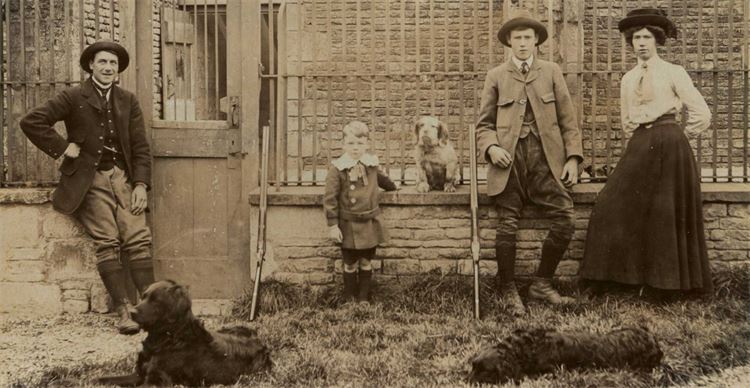The sepia-toned photograph from the early 1900s captures a nostalgic scene of four individuals and two dogs set against a building with an old-fashioned barred steel door. The backdrop features a low brick wall with iron railings. On the far left, a gentleman with a coat, vest, tucked-in boots, and a hat stands near the doorway. Beside him, a young boy dressed in a suit coat, shorts, shoes, and socks stands, accompanied by his dog sitting on a ledge. To the right, a woman in a long skirt, blouse, and hat stands next to another gentleman similarly attired in a coat and tucked-in pants, both looking directly at the camera. In front of them, a large black dog is laying on the ground. The overall image, rich in historical texture, is rendered in various shades of brown and gray, evoking the feel of an era long past.